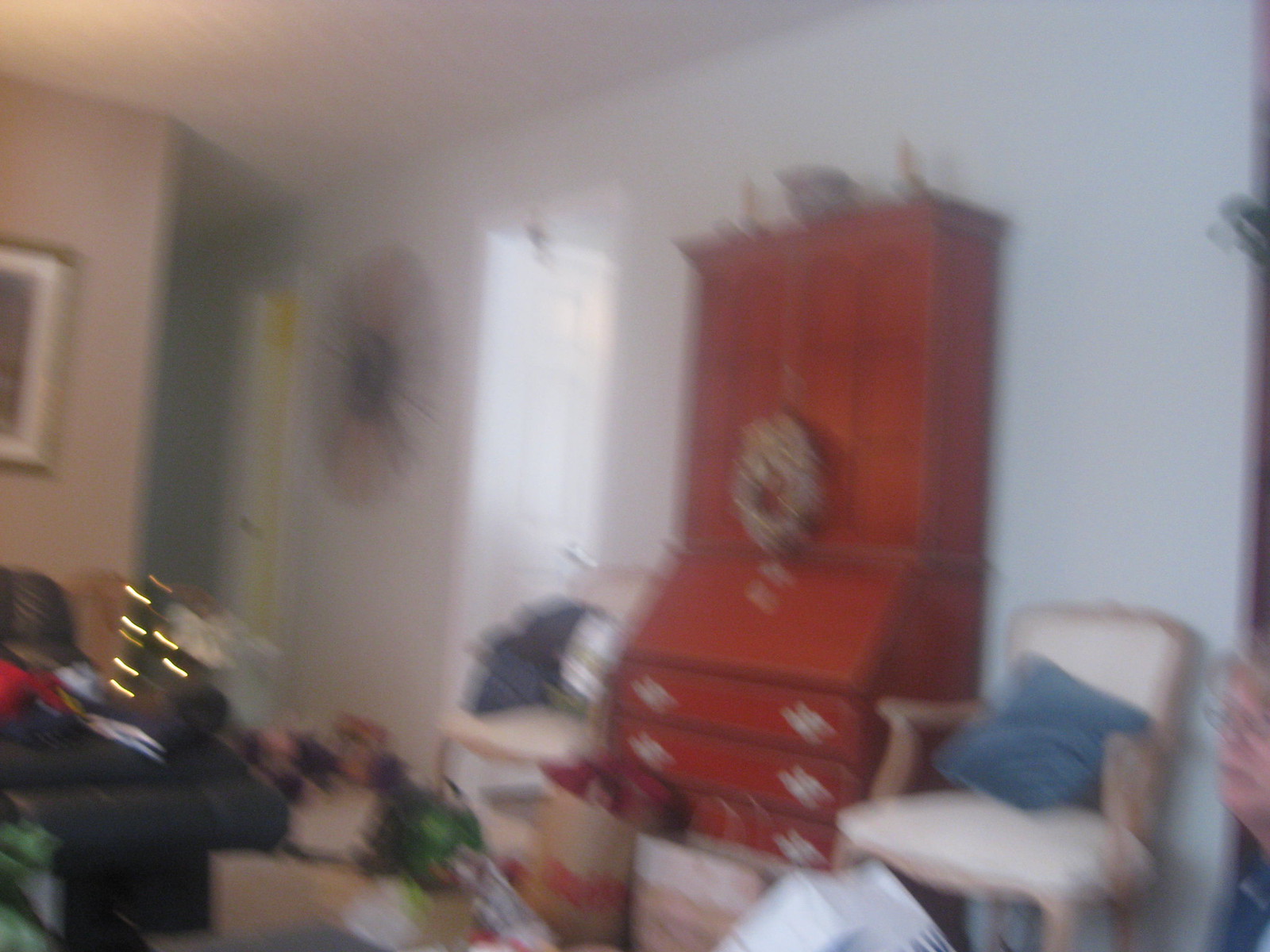In this image, we observe a detailed room setting filled with various objects scattered across the floor. Starting from the right-hand side, the center features a partial side view of a person's face adorned with glasses. To the left of this, the wall is painted in a light gray color. Adjacent to the wall is a blue-cushioned chair. Moving further left, there's a piece of furniture that combines dresser drawers and an upper cabinet-like platform, all in a brown hue. Another blue-cushioned chair is positioned to the left of this furniture. Above these elements, the light gray wall continues.

On the floor, various bags and miscellaneous items spread across, covering the entire floor area. To the far left, part of a green couch is visible, reclined back with chassis, and partially covered by blue and red clothing items.

In the background, on the left side, there's a tan-colored wall featuring the edge of a picture frame and a portion of the ceiling, which is gray.